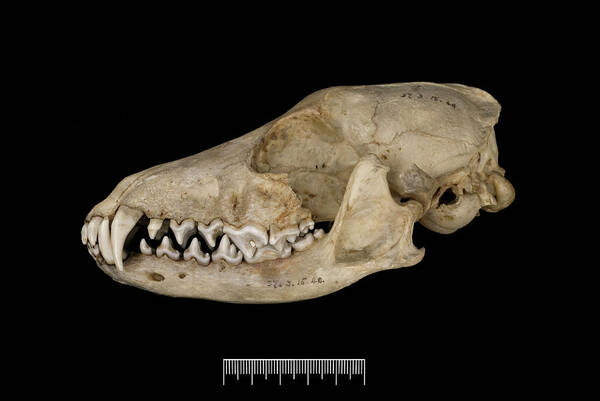This photograph depicts the elongated skull of a Falkland Islands fox, presented against a dark, black backdrop. The skull is prominently white with patches of brownish discoloration. The image captures a side profile view, revealing a notably long snout and large, sharp teeth. Especially prominent are the upper and lower fang-like incisors, one of which extends halfway to the bottom jawline. Intricate details include faint, hard-to-decipher markings on both the jawbone and top part of the skull, potentially reading "57.5.15.4C". Below the skull lies a horizontal ruler marked with white lines of varying lengths, providing scale despite the absence of numerical values.